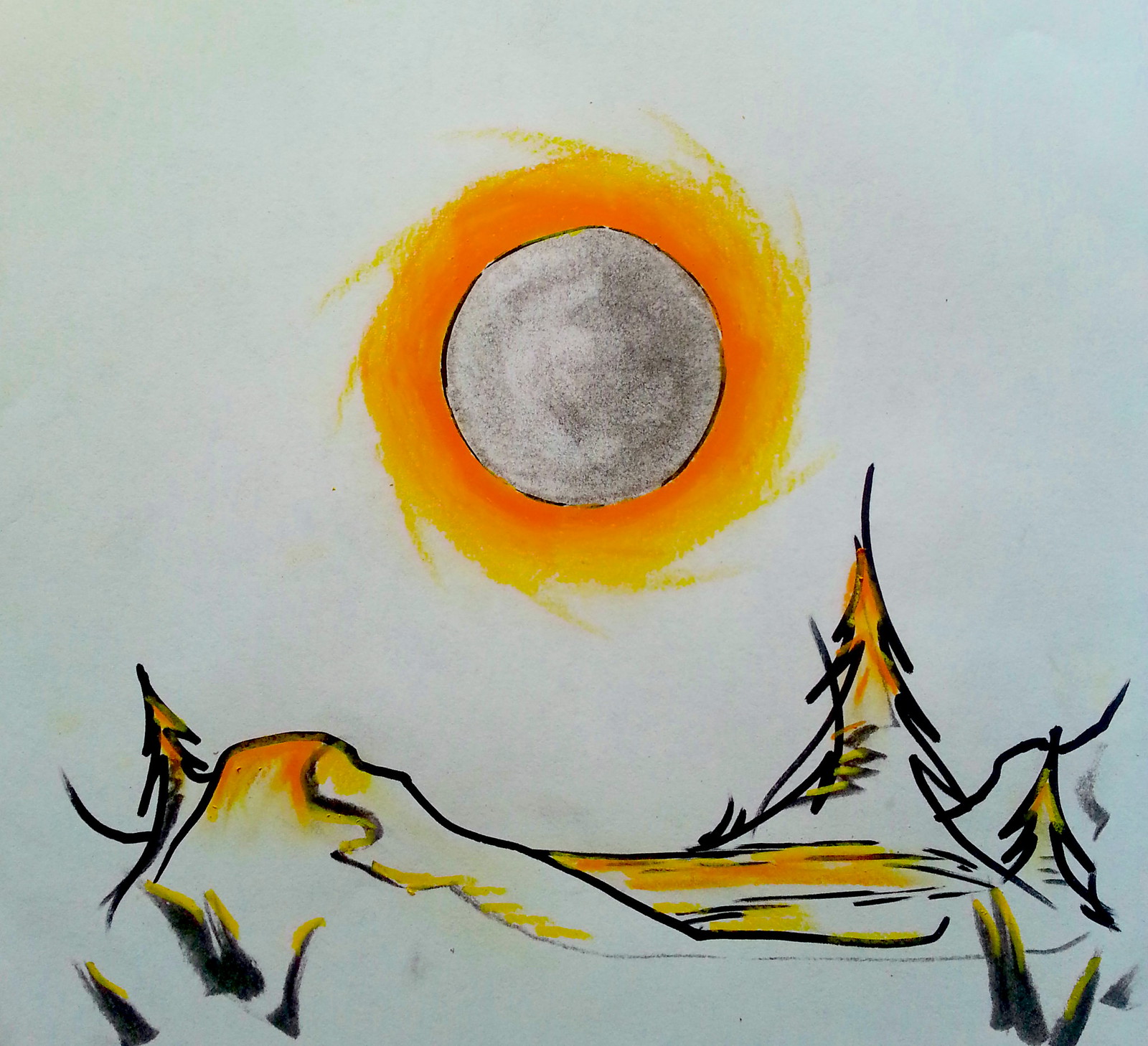The image features a striking drawing on an unidentified surface, possibly done with a marker. The background of the image has a grayish-blue hue. Centrally, near the top, is a prominent circle outlined in black charcoal, filled with a dark, dense shading. Surrounding the circle is a vivid, radiating orange pattern that spirals outward, reminiscent of the intense heat waves emanating from the sun. 

Below this central figure, a landscape of hilly or mountainous terrain spreads out. This landscape is populated with several tall, pointed trees, each resembling the classic shape of a Christmas tree. Of these trees, at least three are prominently visible and are colored orange, suggesting that they may be engulfed in flames, adding a dramatic contrast to the overall composition. The combination of the fiery trees and the heated sun creates a dynamic and intense visual effect.